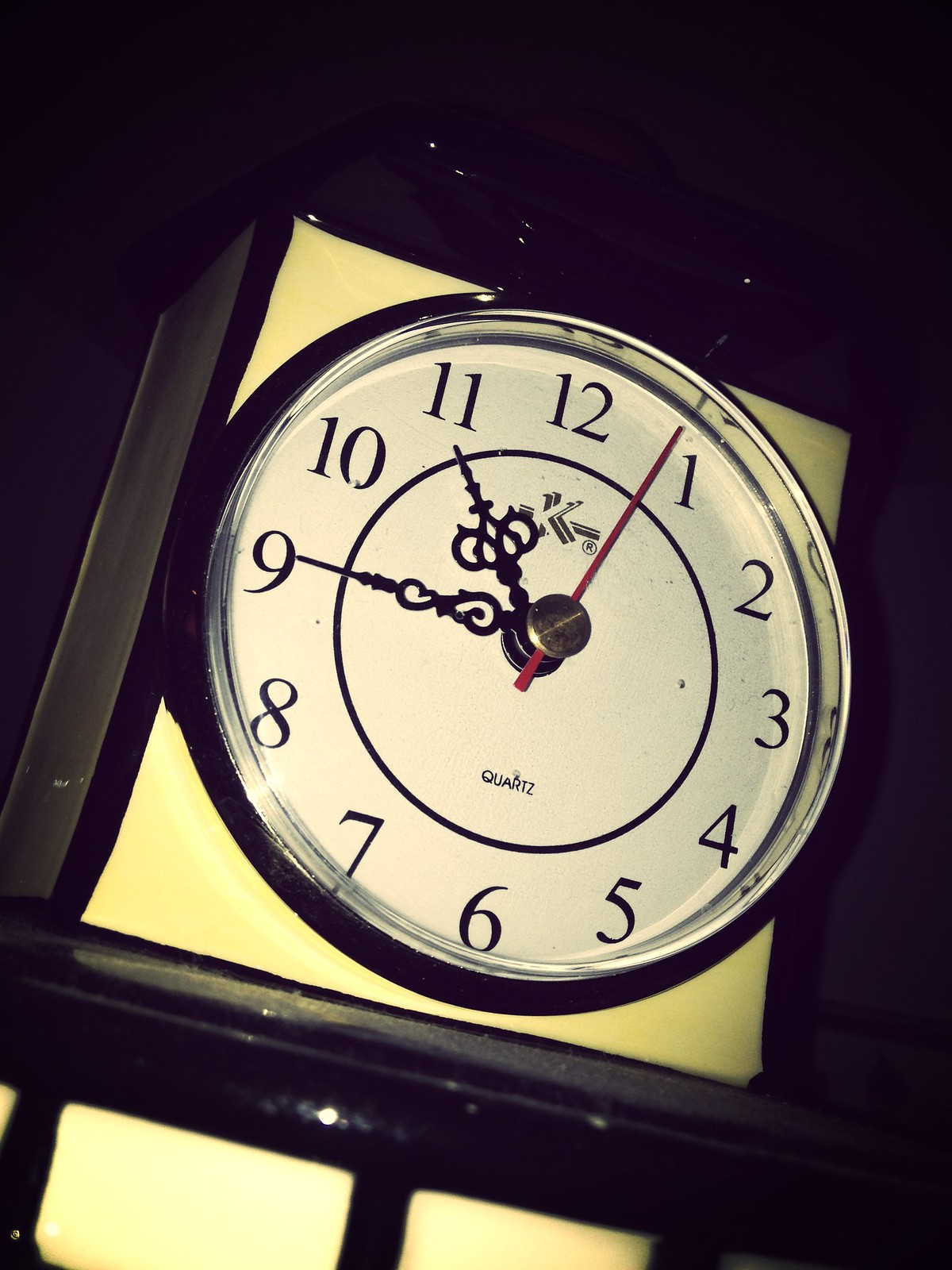A detailed image of an elegant clock featuring a circular face adorned with Roman numerals I through XII. The time on the clock reads precisely 10:45:04. The clock is equipped with an hour hand, minute hand, and a second hand, offering precise timekeeping. Notably, the word "QUARTZ" is prominently displayed just above the numeral VI, indicating the type of movement mechanism used. The clock combines classic design with modern functionality, making it an eye-catching and practical timepiece.